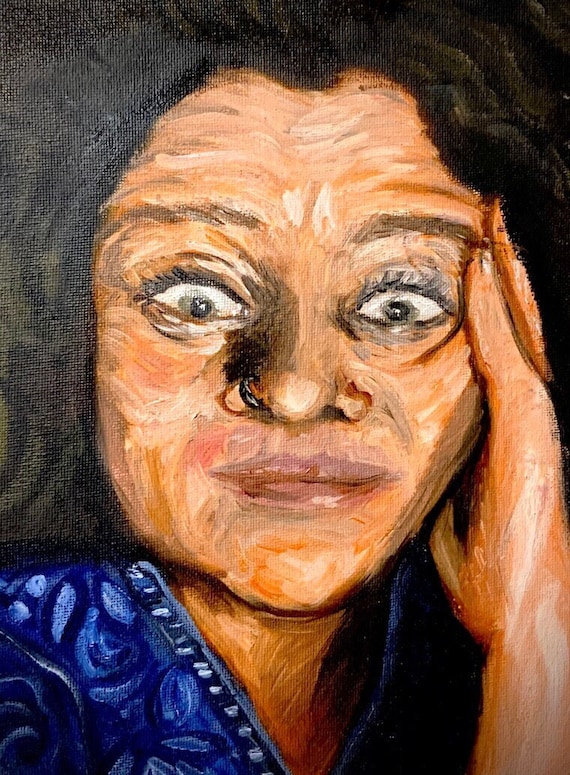The image is a vertically oriented oil painting depicting a woman with a shocked and wide-eyed expression. The painting is created with broad, somewhat smeary brush strokes that give it a less detailed and realistic appearance. The woman, who appears to be advanced in age, has straight black hair, though the length is indeterminate due to the close-up nature of the painting, which captures her face and shoulders. Her left hand is poised alongside the left side of her face near her eyes. She has pronounced wrinkles, indicating her age, and her facial features include wide, slightly downward-looking eyes enhanced with makeup, large lips with lipstick, a wide nose, and a nose ring. Her eyebrows are raised and her mouth is closed in a grimace, with her forehead creased. She is wearing a blue shirt with a v-neck collar. The overall coloration of her skin is light brownish, contributing to the textured, clay-like effect of the painting.